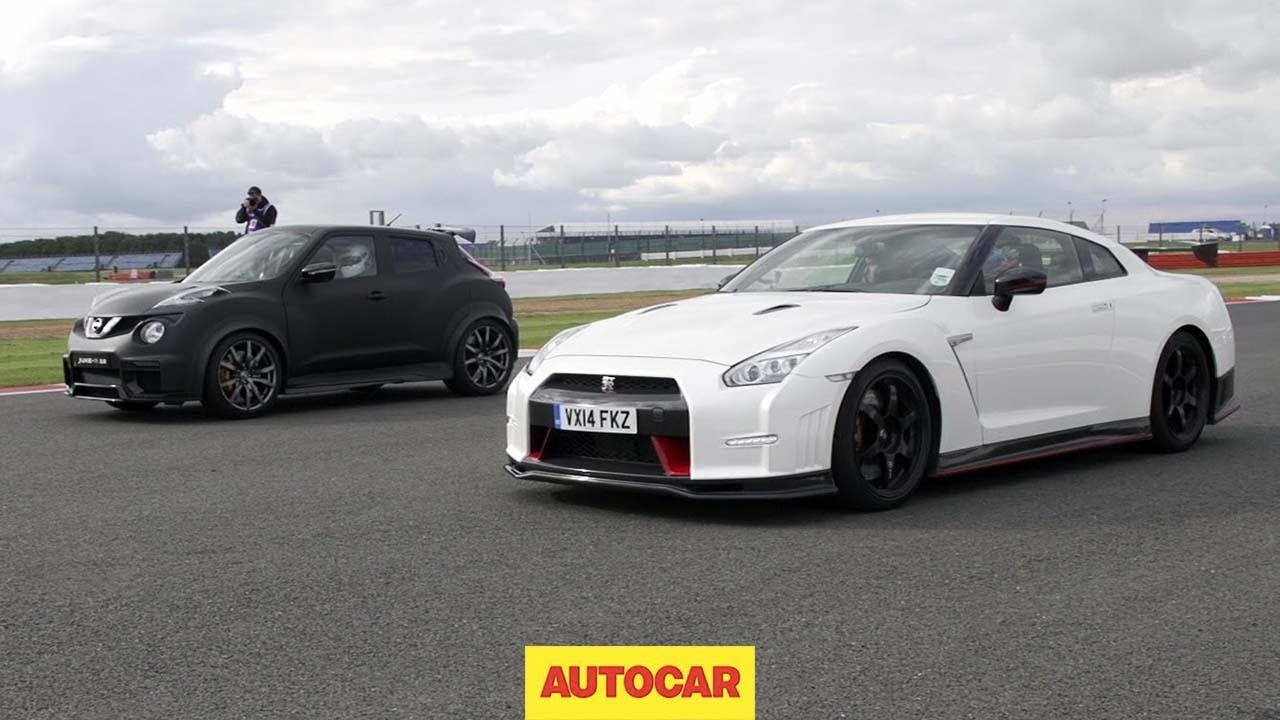The image depicts two distinct vehicles poised on a gray pavement, seemingly ready to race. The vehicle on the left is a matte black Nissan Juke, while the one on the right is a white sports car, likely a Citroën, adorned with black valences and red accents. Both cars house drivers and are facing left. The white car prominently displays a European license plate reading VXI4FKZ. The backdrop features a racetrack with white barriers, green trees, and a red wall with a blue cover on the distant right side. The scene is further detailed with an overcast sky filled with fluffy white clouds, green grass bordering the pavement, and a photographer on the right capturing the moment. At the bottom center of the photo, a yellow rectangle with red text reads "Auto Car."